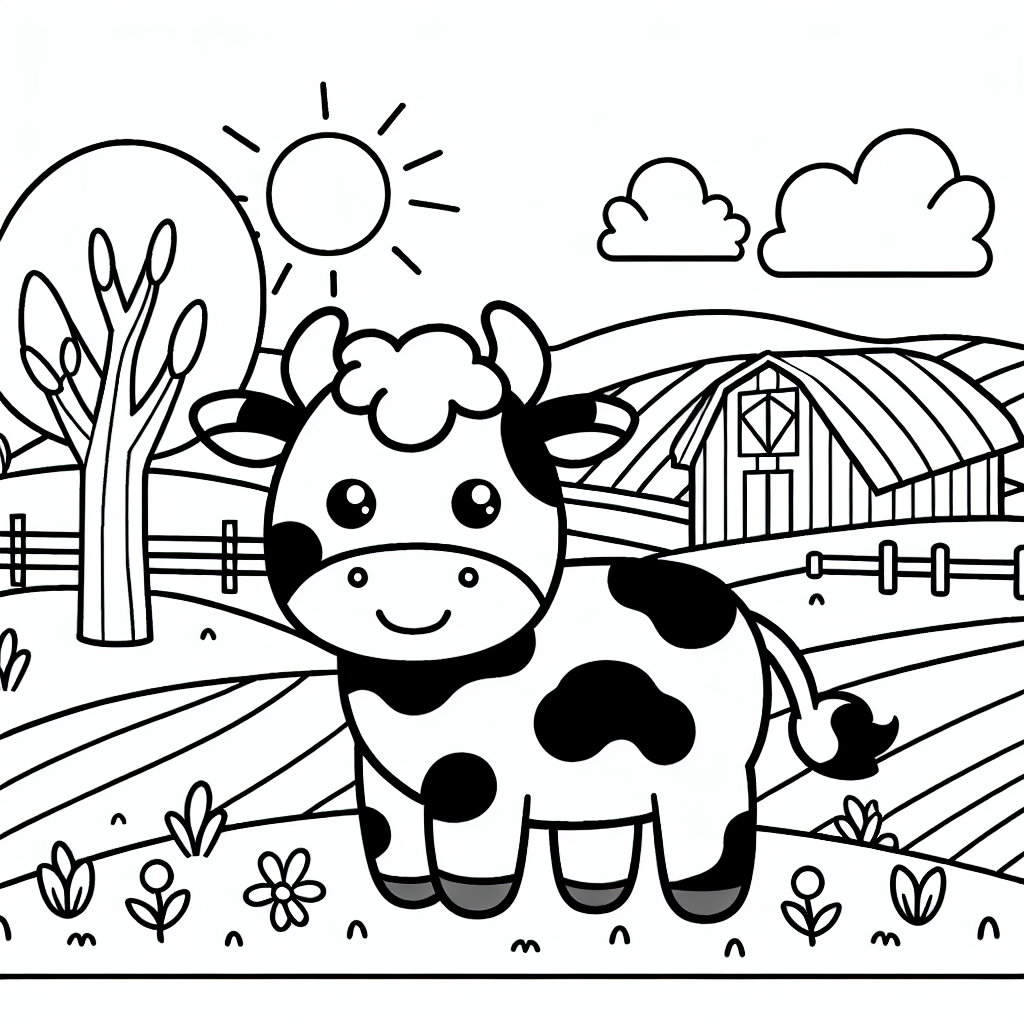This charming black and white illustration, reminiscent of a beginner's coloring book or a child's drawing, depicts a serene farm scene. In the foreground, a friendly, cartoon-like baby cow with big black eyes, black spots, and a tuft of hair on its head stands cheerfully on a hill adorned with flower petals. The cow's endearing smile and tiny horns enhance its adorable appearance. Surrounding the cow are rolling farmlands, characterized by tilled ground with parallel stripes, and a rustic wooden barn situated on the right. To the left, a rudimentary tree with an oval-shaped canopy provides balance to the scene. Above, a round sun with radiating beams and two puffy clouds float in the sky, all drawn with simple, child-like lines. A fence meanders along the left-hand side of the image, adding a sense of depth and continuity to this quaint pastoral setting.